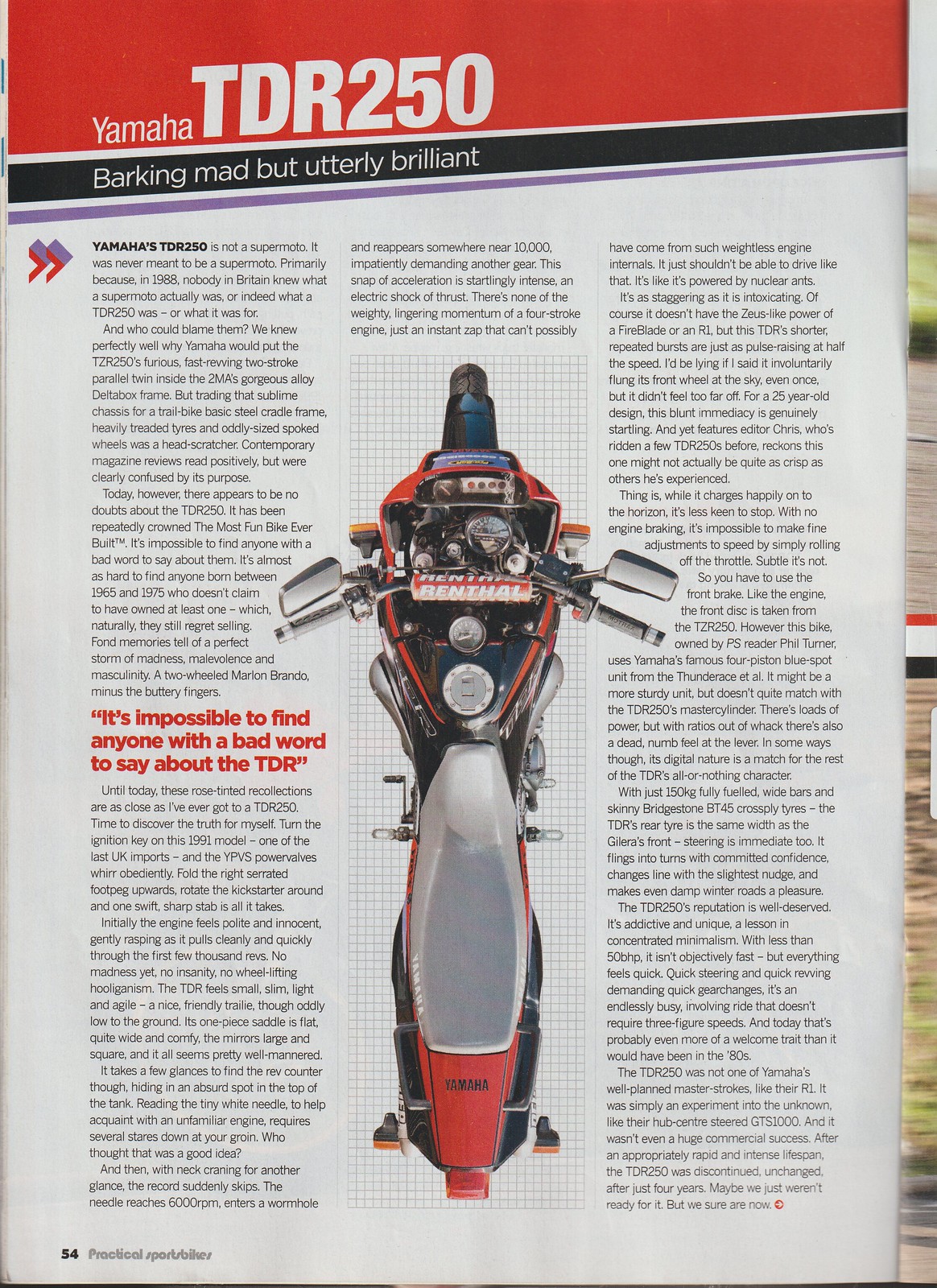The image depicts a magazine page centered on the Yamaha TDR 250 motorcycle. Dominating the page is an overhead photograph showcasing the motorcycle's seat, handlebars, and dash, positioned centrally. The top of the page features a vibrant orange background with bold white text stating, "Yamaha TDR 250." Directly beneath, within a black box, another statement reads, "Barking Mad, but Utterly Brilliant." Flanking the photograph, long columns of text provide detailed information about the TDR 250, although some text is difficult to read. A standout quote in larger, red letters on the left column asserts, "It's impossible to find anyone with a bad word to say about the TDR." The bottom left corner of the page notes the page number, likely "54," and refers to Practical Sports Bikes magazine. The color scheme interlaces red, black, and other shades throughout the layout, complementing the technical yet enthusiastic tone of the page.